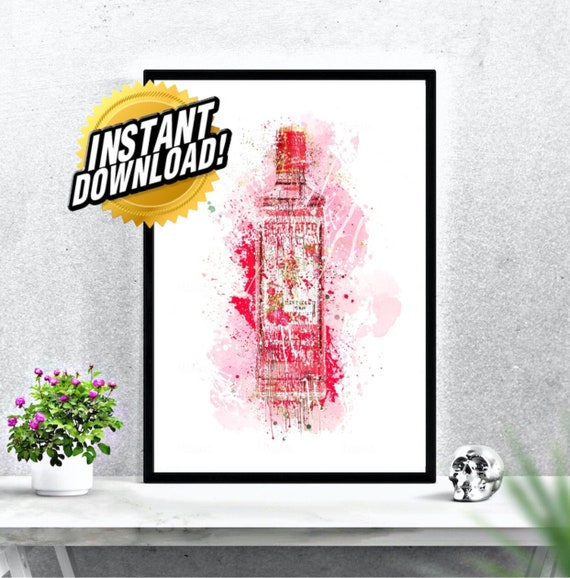The image is a stock photograph featuring a stylized painting of a Beefeater liquor bottle, rendered in red and pink hues with paint splatters and drips, creating a messy, abstract effect. This artwork is propped up on a white-gray table against a grayish-white wall, and is framed in black. Superimposed on the left side of the painting is a gold seal with the text "instant download" in white letters outlined in black. To the left of the framed painting, there is a white vase filled with purple flowers and green foliage, adding a natural touch to the scene. On the right side of the table, there is a silver-colored skull, adding an eclectic element to the composition. The table itself has a marble-like appearance, completing the modern aesthetic of the setup.